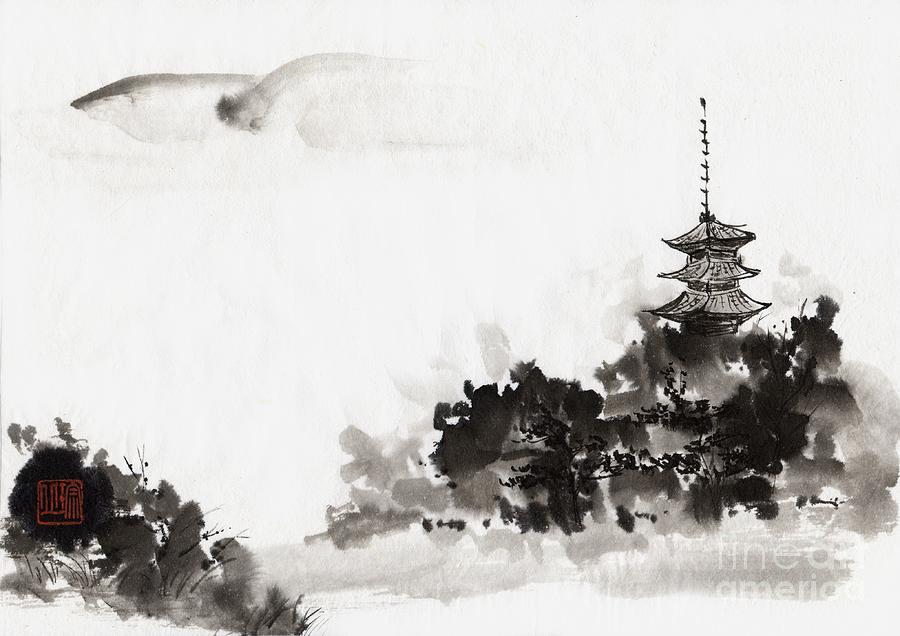This black and white watercolor painting depicts a Japanese-style pagoda with three cascading roofs, each progressively larger as they descend. The topmost tier is the smallest, followed by a medium-sized roof in the middle, and the largest at the base. The building is set against a backdrop of dense, impressionistic blotches that resemble either lush, towering foliage or clouds of smoke, creating a sense of depth and mystery. The sky remains mostly clear, contributing to the overall minimalistic and evocative feel of the artwork. In the bottom right corner, faint and barely legible words appear to read "Sign America," though the full text is indistinct.